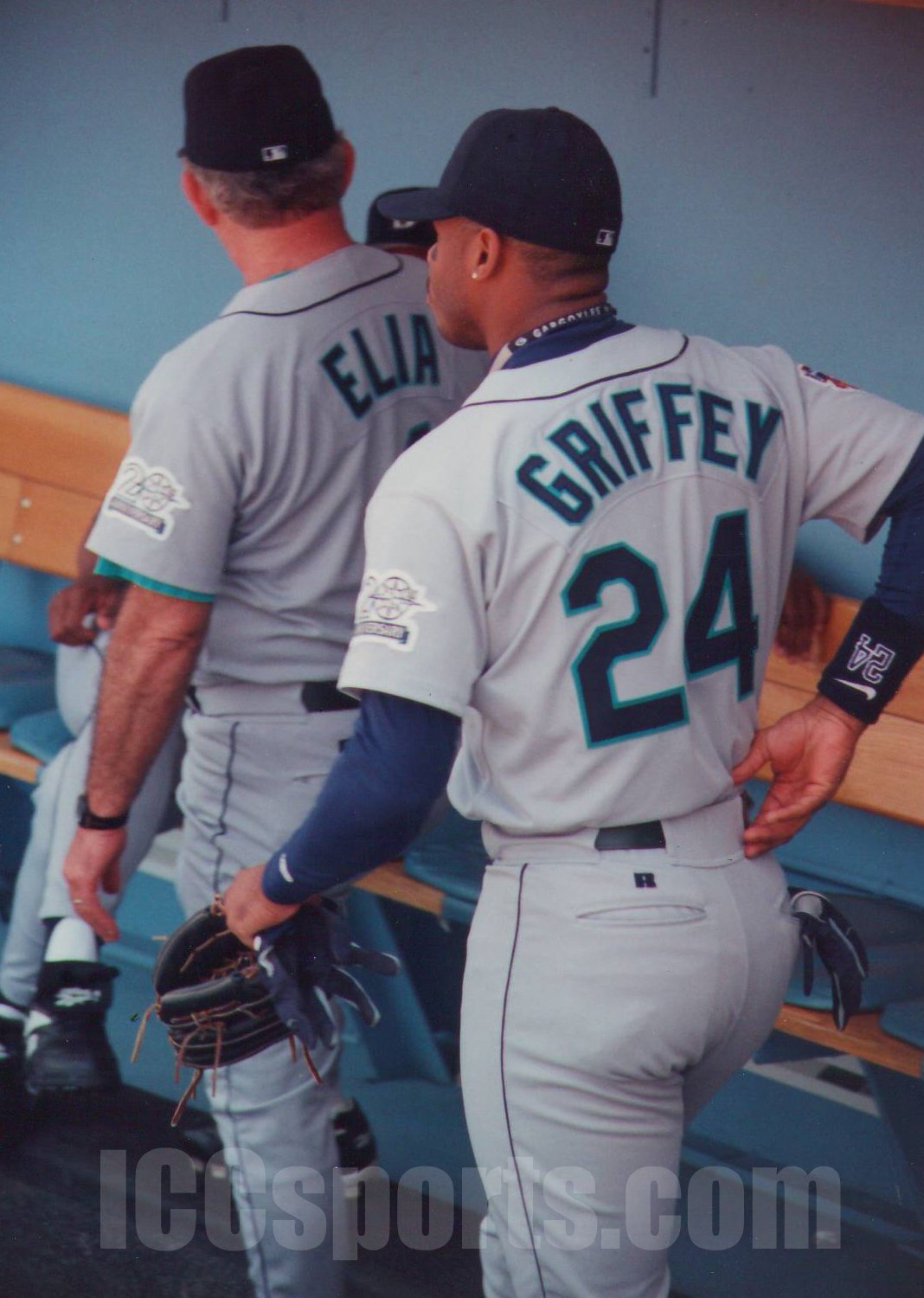This photograph captures two baseball players in a dugout, one of whom is the iconic Ken Griffey Jr., recognized as one of the greatest players of all time. Ken Griffey Jr., donned in his Seattle Mariners uniform with the number 24 on the back, stands with his back turned to the camera. He's wearing a black baseball cap and a sweatshirt under his jersey, and his right hand is reaching behind him towards his belt while his left hand holds a loosely-strapped mitt. In front of him, another player or possibly a manager, whose shirt has "Aliyah" written on it, faces towards the top left corner. The scene is set in an outdoor stadium, characterized by the light brown benches of the dugout and a color palette featuring black, teal or aqua, and white.